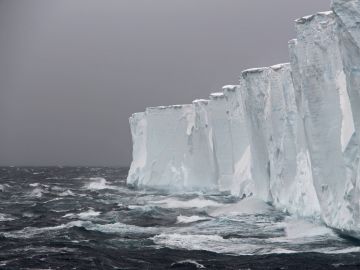The monochromatic photograph captures the immense and stark beauty of an ice shelf stretching out from the right side and extending to just past the image's center. Towering hundreds of feet high, this formidable shelf of ice has a flat top and a wavy, textured front face that meets the sea. The sea, a turbulent gray-green expanse, crashes its waves forcefully against the ice, highlighting the scene's raw and untamed nature. The ice itself is an intricate blend of pristine white interspersed with streaks and patches of gray, showcasing the complex interplay of light and shadow. Above, a dark gray, cloud-laden sky looms, adding a foreboding ambiance and accentuating the desolate beauty of this frozen wilderness.